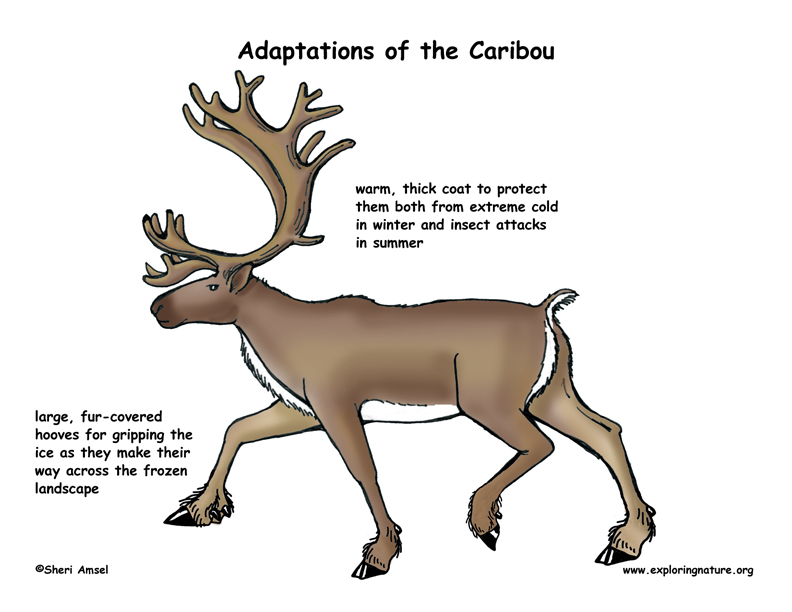The image is a detailed, somewhat cartoony drawing of a caribou, also known as a reindeer. At the top of the illustration, the text reads "Adaptations of the Caribou." The caribou is depicted with very long, massive curved antlers that have branch-like structures extending from them. It has a brown body with a white underbelly and a small tail. The descriptions in black text on the image highlight key adaptations: a warm thick coat to protect the animal from extreme cold in the winter and insect attacks in the summer, and large, fur-covered hooves for gripping ice as they traverse the frozen landscape. The bottom left corner of the image contains the artist's name, Sherry Amsel, along with a copyright notice, and the bottom right corner includes the website exploringnature.org.